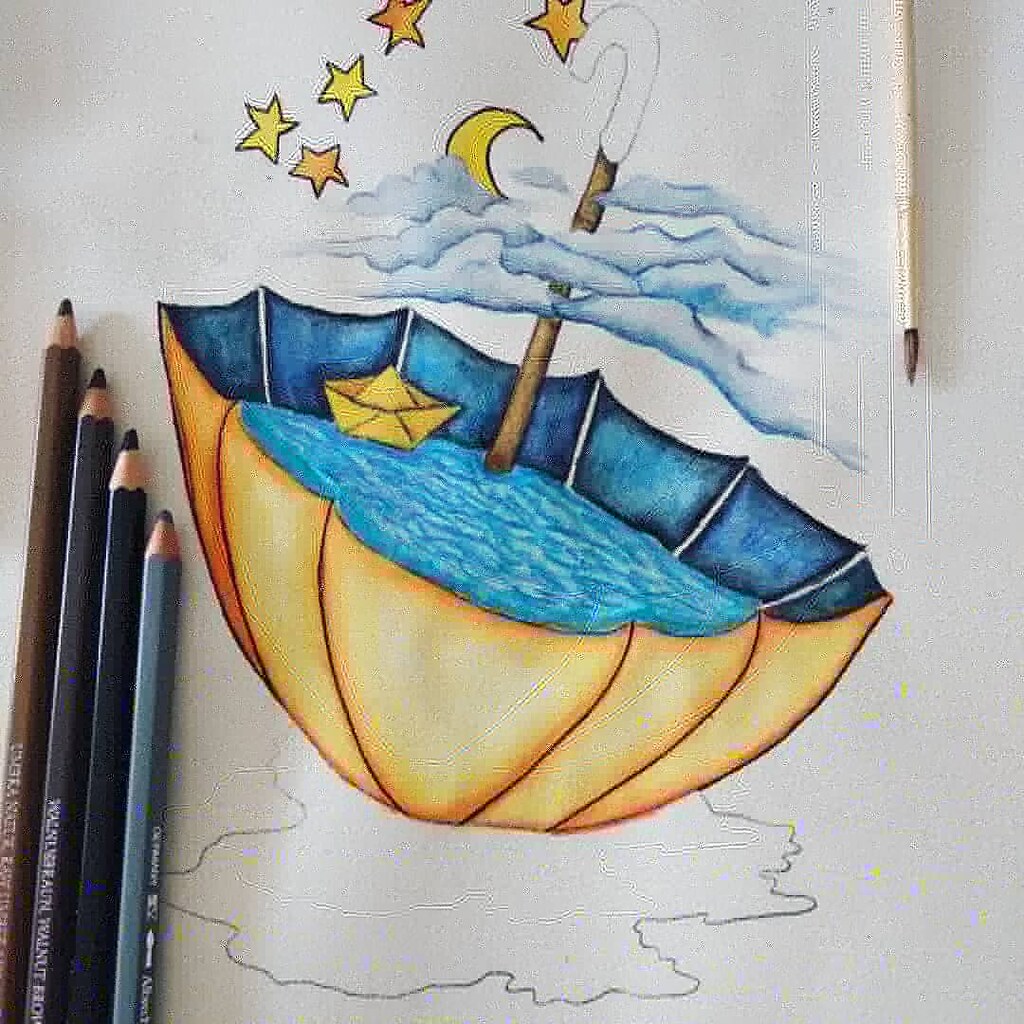This is a detailed color pencil illustration captured in a photo, with some watercolor elements perceptible. The artwork is on a sheet of white paper, featuring an upside-down umbrella with a white-tipped, brown, wooden-finished handle. The inside of the umbrella is colored blue, depicting pooled water with a folded yellow toy boat floating in it. The exterior of the umbrella is a yellowish-golden hue. Surrounding the umbrella's water-filled basin, there's an uncolored puddle, indicating it's still a work in progress. Above the umbrella's handle, the sky contains light blue clouds, along with a crescent moon and vibrant orange and yellow stars. The composition is complemented by four color pencils and a paintbrush placed on the upper right side of the paper, hinting at the ongoing creative process.